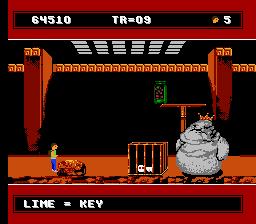This screenshot captures an old-school side-scrolling game, likely from the Super Nintendo era, which many believe to be "A Boy and His Blob." The setting features a dark, dungeon-like warehouse with an orange hue, and a protagonist boy in a green shirt and blue jeans. To his right is a rock and a cage containing a small white creature, possibly the boy's blob companion. Confronting the boy is a large, menacing gray blob creature adorned with a crown, exuding a villainous aura. The heads-up display includes the score “64,510” at the top, with “TR = 09” below it, an icon with a “5” indicating lives, and at the bottom, the text "LIME = KEY" in capital letters.